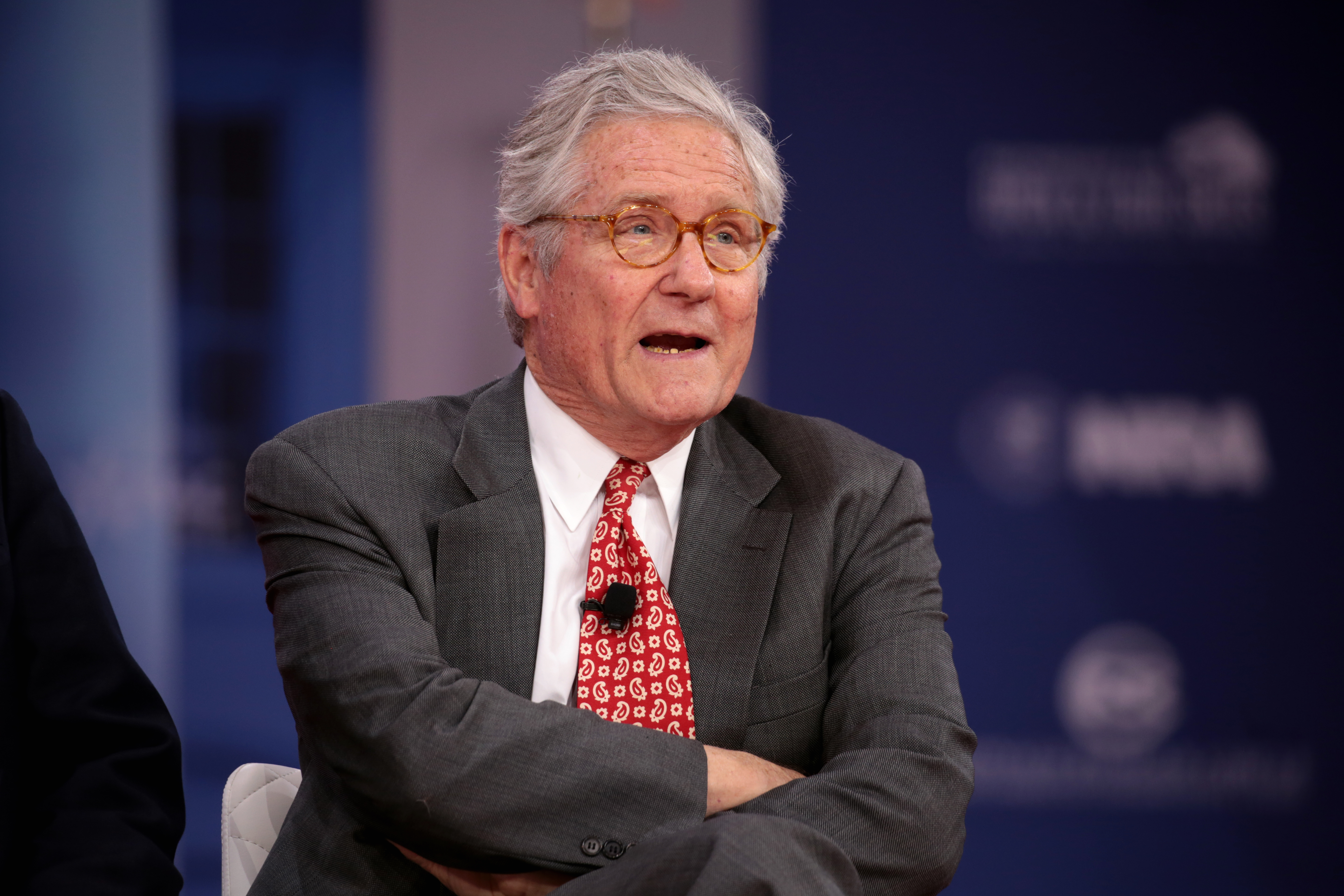This is a detailed photograph of an older Caucasian male political commentator seated in a studio. He is wearing a gray suit, white shirt, and a red tie adorned with a white paisley-like pattern. The man has short to medium-length gray hair, circular brown glasses with clear lenses, and visible signs of aging such as wrinkles and sunspots. His posture is notably crossed, with both his arms and legs crossed, as he appears to be mid-speech with his slightly open mouth exposing a glimpse of his crooked teeth. A black microphone is clipped to his tie, and he is seated in a white chair against a predominantly blue and white studio background. There might be another person partially visible to the left, discernible only by an arm. The photograph is slightly wider than it is tall.